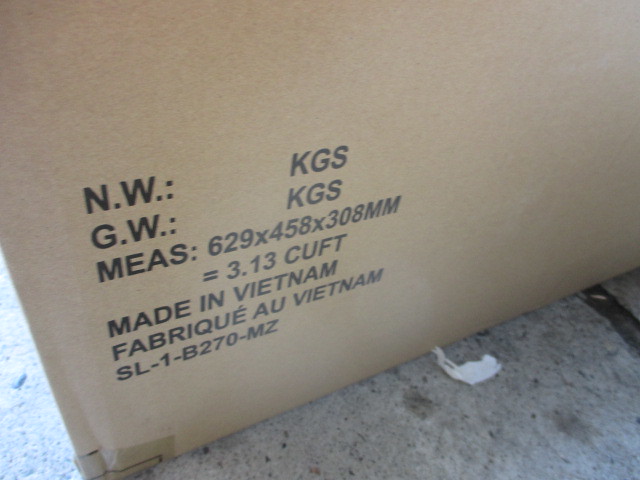The photograph shows a brown cardboard box partially captured, positioned diagonally with its lower left-hand corner visible. The box rests on an unpolished, gray cement floor that features a bumpy texture, scattered rocks, and areas stained with gray and tan dirt. Additionally, a piece of white paper or tape lies at the bottom of the box. The visible surface of the cardboard is marked with black printing that reads: "NW KGS, GW KGS," and "MEAS 629 by 458 x 308 mm = 3.13 CUFT." Other text includes "Made in Vietnam," "Fabrique au Vietnam," and the code "SL-1-B270-MZ." The box’s net weight area for kilograms is currently blank, indicating it has yet to be filled in, likely at the factory.